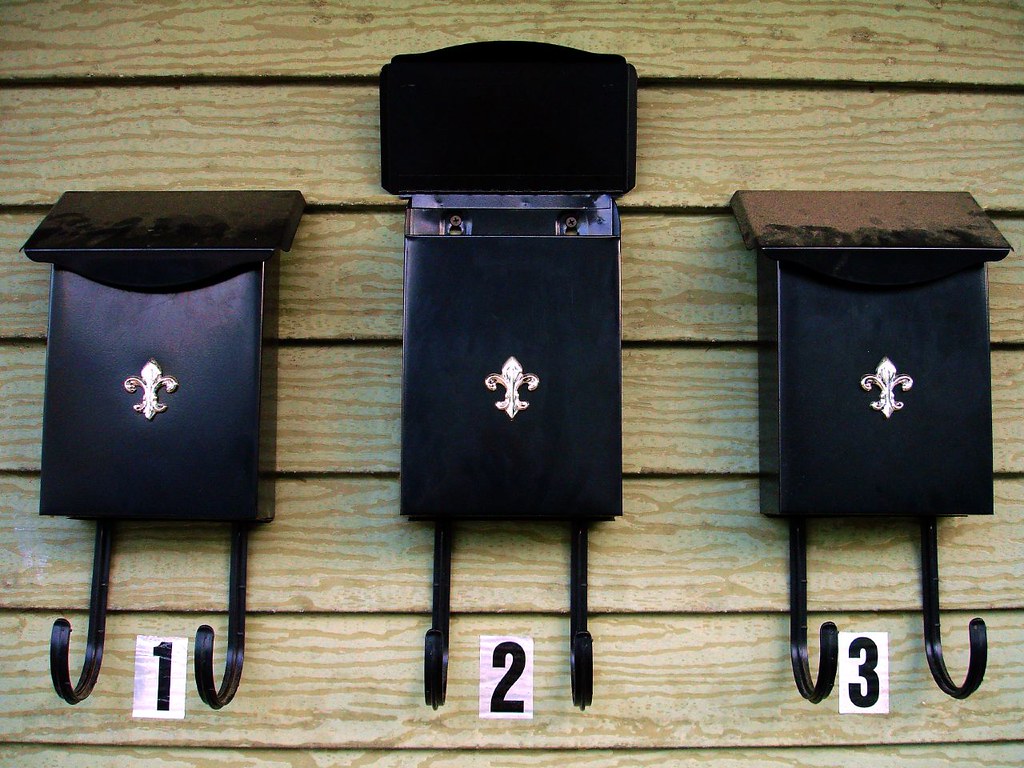This photograph captures the side of a house with a light-colored wooden wall featuring three wall-mounted mailboxes, labeled consecutively from left to right as 1, 2, and 3. Each mailbox, crafted from black metallic steel, sports a similar design with a hinged flap at the top for letter insertion. Prominently displayed on the front of each box is a reflective silver fleur-de-lis emblem. Below each mailbox, there are J-shaped hooks presumably intended for holding packages or bags. Notably, the middle mailbox is open, revealing an empty interior. The rightmost mailbox shows signs of age and wear, with a rusty, dust-covered lid, a contrast to the other two mailboxes. These mailboxes are evidently part of a multi-unit dwelling, given their uniform appearance and close arrangement.